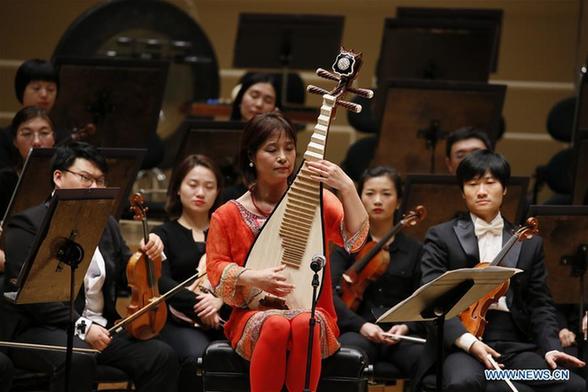In this color photograph, a concert scene unfolds with an Asian woman dressed in a striking red outfit as the central figure. She is holding an ancient-looking string instrument on her lap, which resembles a blend of a lute, mandolin, and a cello, and is played with her fingers. The woman, with short black hair, is seated in front of a microphone and a music stand, intently looking at the sheet music. Surrounding her are fellow Asian musicians; the men are dressed in black jackets with white shirts and white bow ties, while the women don black dresses. Each musician has a violin resting on their lap and is looking down, some with eyes closed, in a solemn, concentrated stance. There are numerous music stands scattered among them, and in the background, a doorway is visible, further enhancing the ambiance of this evocative orchestra performance. The bottom of the image reads "news.cm".